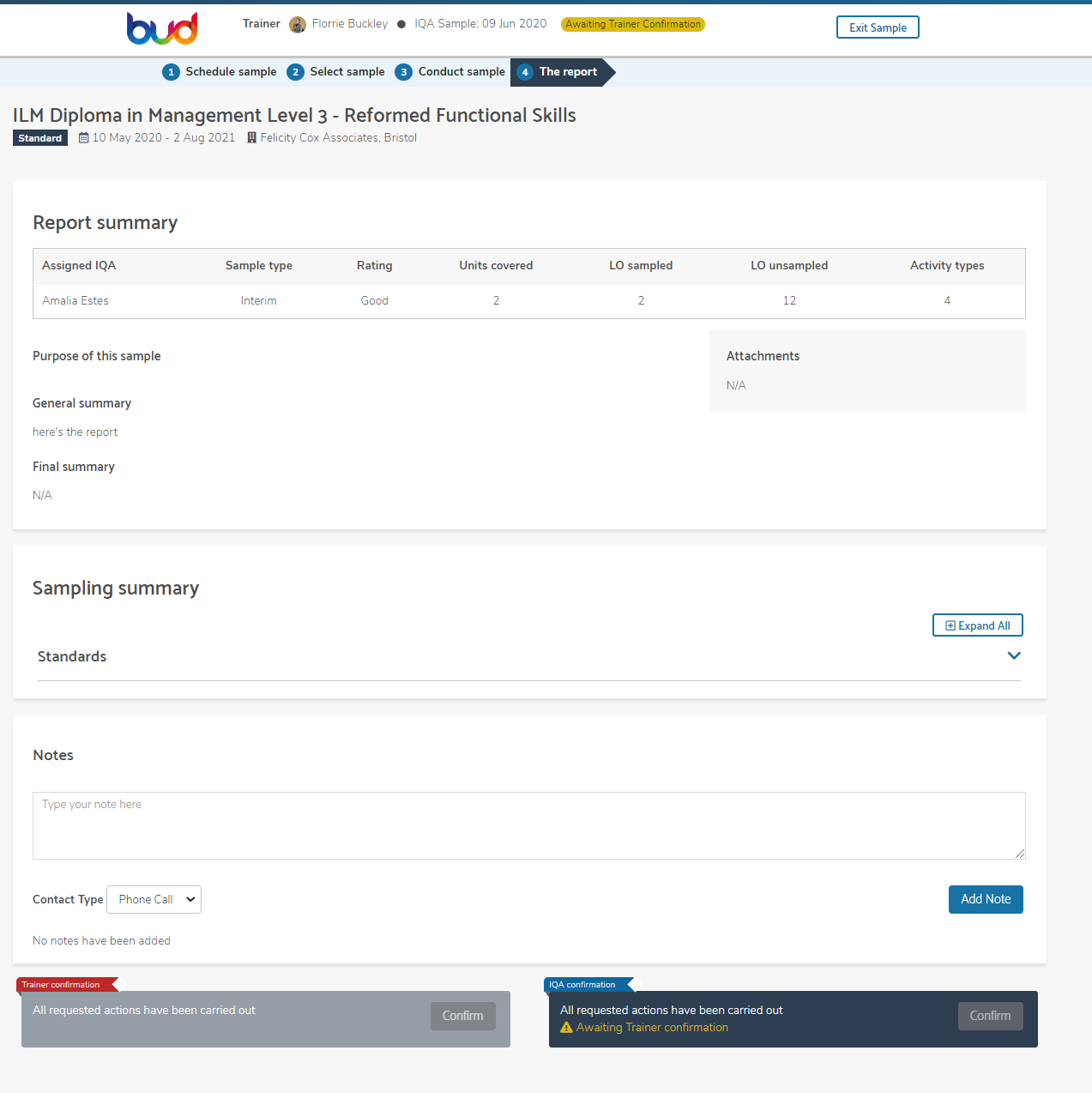In this screenshot of the website BUD, the upper left corner prominently displays the BUD logo adorned in rainbow colors. To the right, the page identifies a trainer named Fiorn Buckley, accompanied by a small profile image. Adjacent to this, the text "IQA Sample, 9th of June 2020, Awaiting Trainer Confirmation" is displayed. 

Nearby, a small white box labeled "Exit Sample" is visible. The interface below features a sequence of options from left to right: "Schedule Sample 1, 2nd," "Select Sample," and "Conduct Sample 3," culminating in a black box labeled "For the Report."

In bold black text beneath these options, the caption reads "ILM Diploma in Management, Level 3, Reformed Functional Skills." Following this, the timeframe "10th of May 2020 through 2nd of August 2021, Felicity Cox Associates, Bristol" is highlighted. The lower section of the page comprises headings such as "Report Summary," "Purpose of this Sample," "General Summary," and "Final Summary."